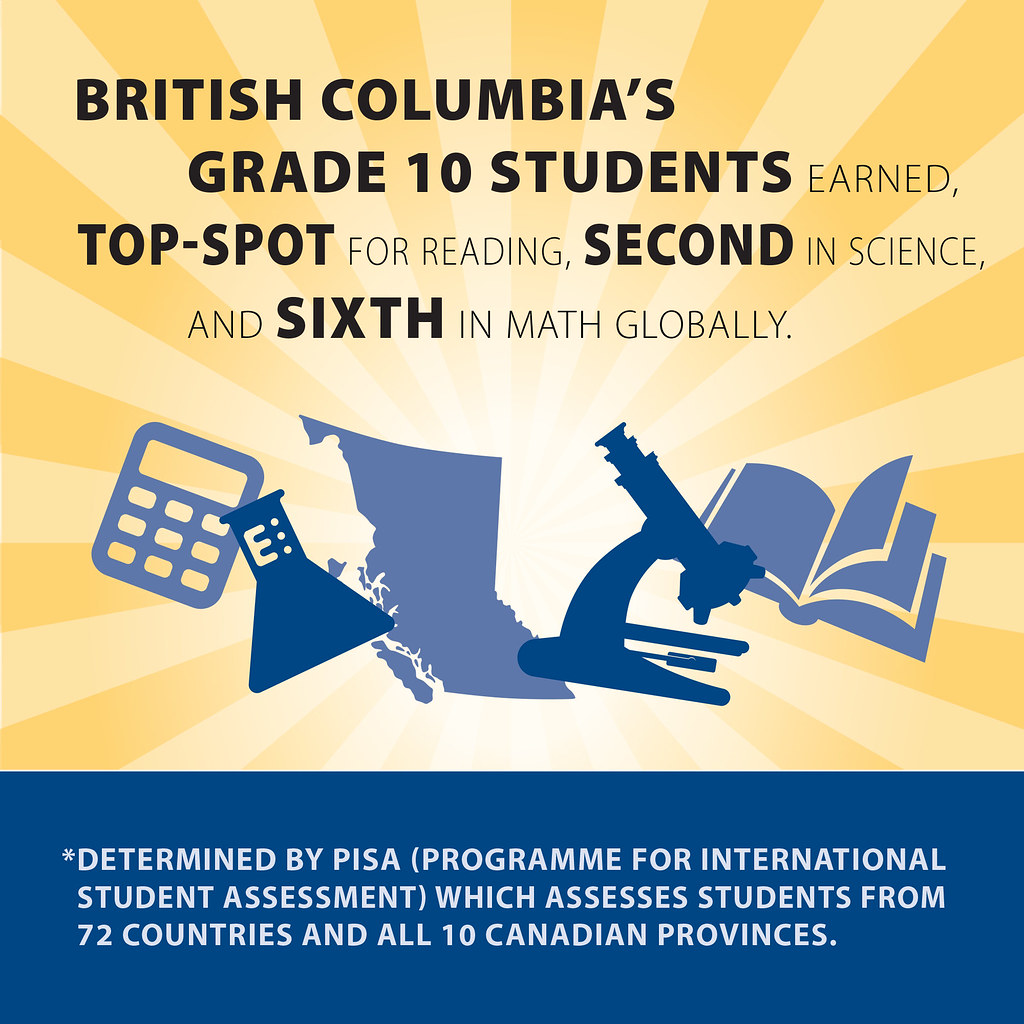The image is a promotional poster highlighting the achievements of British Columbia's grade 10 students on an international scale. The design features a vibrant yellow and blue color scheme, with the top 80% primarily yellow transitioning to white in the center, giving the impression of a sunburst. This pattern radiates outward and fades into perspective toward the bottom. 

Overlaying the sunburst are blue silhouettes of educational tools, including a calculator, a map of British Columbia, a flask, a microscope, and an open book, symbolizing the resources and subjects these students excel in. Above these symbols, black text proudly states, "British Columbia’s grade 10 students earned top spot for reading, second in science, and sixth in math globally." 

The bottom quadrant of the poster is a solid blue block with white text that includes an asterisk, providing additional context: "Determined by PISA, Program for International Student Assessment, which assesses students from 72 countries and all 10 Canadian provinces." This detailed information underscores the global context of the students' achievements.